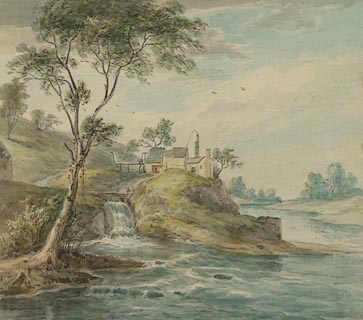The image is a small, detailed illustration seemingly created with colored pencils, characterized by its subtle, soft hues. The centerpiece is a serene stream flowing gently through a valley, fed by a small, graceful waterfall. On the riverbank, a lone tree, which appears to be somewhat withered yet still adorned with green leaves, stands as a sentinel next to the water. The water itself, depicted in shades of blue with delicate ripples and white rapids, winds its way through the landscape, flanked by grassy hills and scattered trees.

On one of the hillsides, slightly elevated, there is a quaint house with a yellowish facade and a black roof, alongside what appears to be a barn and a silo. The house is surrounded by rocky outcrops and patchy greenery, suggesting a rugged terrain. The hillside extends further to reveal additional scattered trees.

The sky above is a blend of muted blue, gray, and white, with soft, airy clouds and a few birds flying across. Though the colors throughout the scene are light and occasionally faded, they evoke a calm, pastoral atmosphere, emphasizing the peaceful seclusion of the countryside setting.